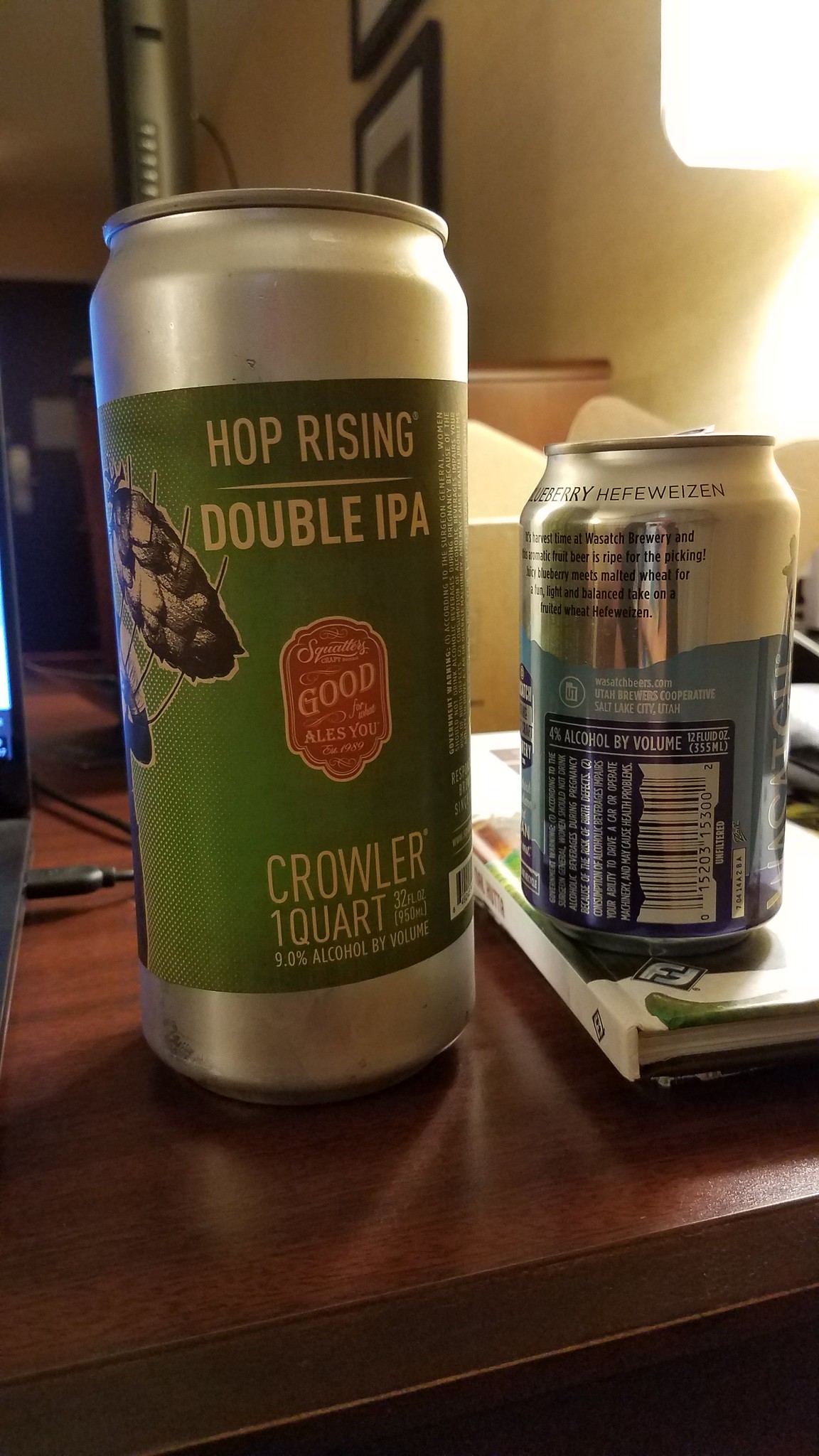In the image, two aluminum cans are prominently displayed on a brown table in a living room setting. The can on the left is tall, silver, with a prominent green label that says "Hop Rising Double IPA" in white text. It also includes red and white details, and appears to feature a drawing of a horse on the front. Additional text such as “crawler” and “one quart” is visible, with a distinct red oval marking the word "good" near the middle of the can. To the right, a shorter can is positioned on top of a white book, displaying its back with visible nutritional facts and ingredients. The shorter can is white, silver, and blue in color. The background reveals a white wall adorned with several framed pictures, which have either brown or black frames, adding a homey ambiance to the scene.